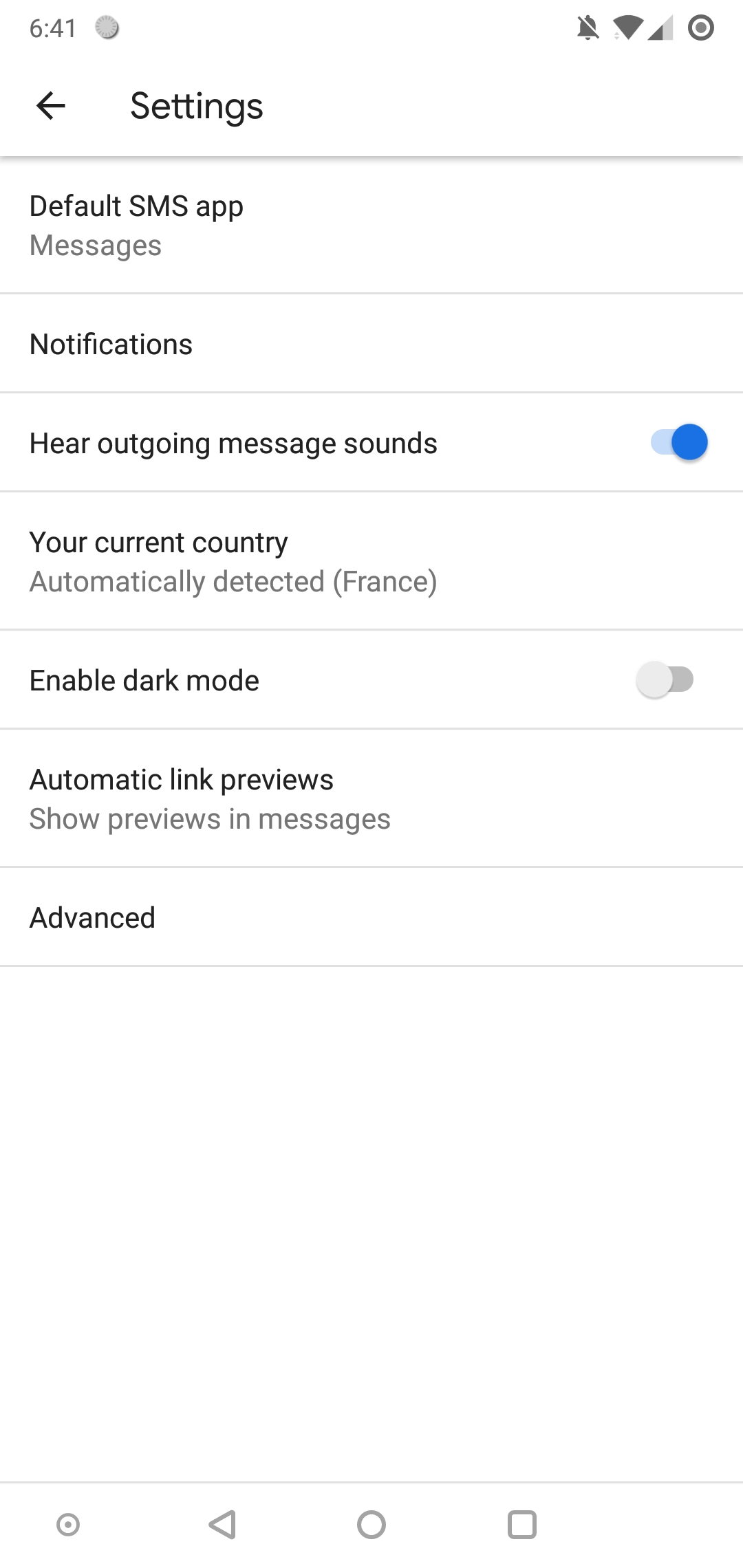**Descriptive Caption:**

The image is a detailed screenshot of a smartphone's settings page, featuring various configuration options. The background is white with black text, and at the top of the screen, the word "Settings" is prominently displayed in black, accompanied by a black back arrow. Notable icons on the status bar include a sun symbol indicating a heat warning, a silent mode icon showing the phone's sound is muted, Wi-Fi connectivity at full strength, cellular reception at about half strength, and active location services. The battery status is not clearly visible.

Key settings displayed include the "Default SMS App" set to "Messages," and a section on "Notifications." Within this section, the option for "Outgoing Message Sounds" is highlighted and selected. The current country is automatically detected as France. The option to enable dark mode is turned off. Additional settings like "Automatic Link Previews" for short previews of messages and an "Advanced" settings section are also visible.

At the bottom of the screen are standard navigation buttons: a power button, back button, home button, and a context menu button. In the background, partially visible, is a dog, presumably belonging to the owner of the phone.

The settings page captured in this image showcases essential configurations and notification preferences for the device, which could be a phone or a tablet.